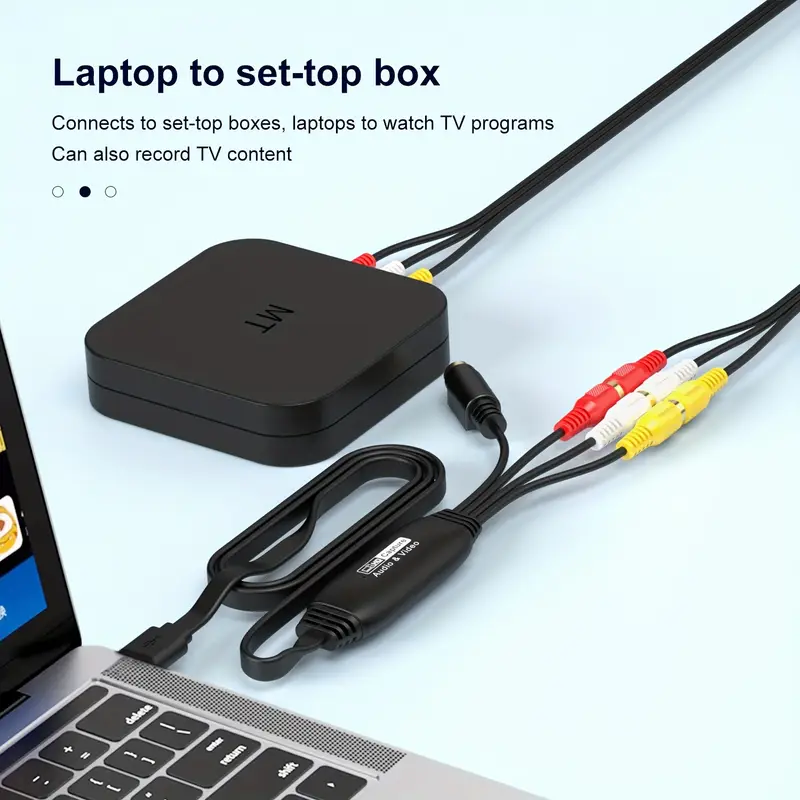The image showcases a professional advertisement of a small, black electronic device designed for connecting a laptop to a set-top box, allowing users to watch and record TV programs. Set against a light blue backdrop, the scene is a close-up, revealing the connections and components in detail. The black box, labeled "MT," features red, white, and yellow audio-video cables, indicative of standard AV inputs—the red and white for audio, and the yellow for video. The device connects to an Apple laptop, identifiable by its silvery color and black keys, through a USB port. The text at the top reads "Laptop to Set-Top Box," with smaller text detailing its functionalities: "connects to set-top boxes, laptops to watch TV programs, and can also record TV content." Additionally, three circles are depicted, with the central one filled in black, suggesting overlapping sets of information or functionalities. The photograph provides a comprehensive visual guide on how to establish the connection between the laptop and the set-top box, highlighting the practical use of the black device and its accompanying cables.